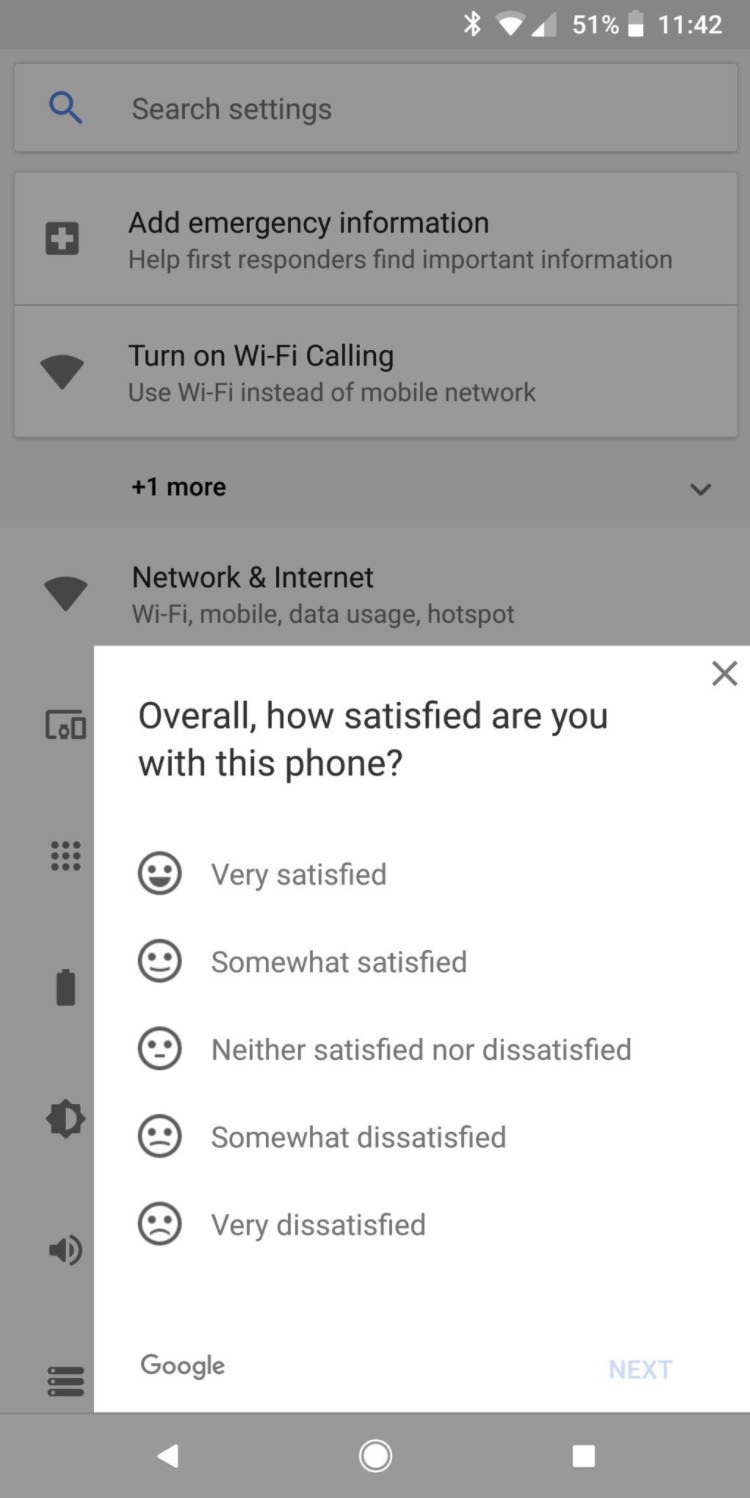In the background of the image, we see a mobile phone's settings screen, largely grayed out to emphasize the pop-up box in the foreground. The background shows that the phone has Bluetooth enabled, Wi-Fi connected, strong signal strength, approximately 51% battery life, and the time displayed is 11:42. Various settings options are partially visible, including icons and text details. The first icon is a blue magnifying glass labeled "Search settings," followed by a first aid sign that says "Add emergency information, help first responders find important information." Further options include "Turn on Wi-Fi calling" and a drop-down labeled "Plus one more.” Additional visible settings categories include "Network and internet," featuring Wi-Fi, mobile data, usage, and hotspot sections, along with icons for a computer, tablet, and watch. Other icons indicating different settings are arranged vertically: a square made of nine dots, a battery icon showing full, an icon for light and dark modes, and icons for screen brightness and sound controls. Lastly, an icon with three horizontal sliders is noticeable at the bottom.

In the foreground, the focus is on a bright pop-up box that prominently asks, "Overall, how satisfied are you with this phone?" The box presents five satisfaction options: a very happy face labeled "Very satisfied", a smiley face labeled "Somewhat satisfied", a neutral face labeled "Neither satisfied nor dissatisfied", a somewhat sad face labeled "Somewhat dissatisfied", and a very sad face labeled "Very dissatisfied". Each option has an accompanying facial expression icon. At the bottom part of this pop-up, there’s a label "Google" and a "Next" button, which is grayed out and currently unclickable. In the bottom navigation bar of the phone, typical navigation buttons are visible: a white triangle pointing left, a circle with a white center and border, and a white square, all set against a gray background.